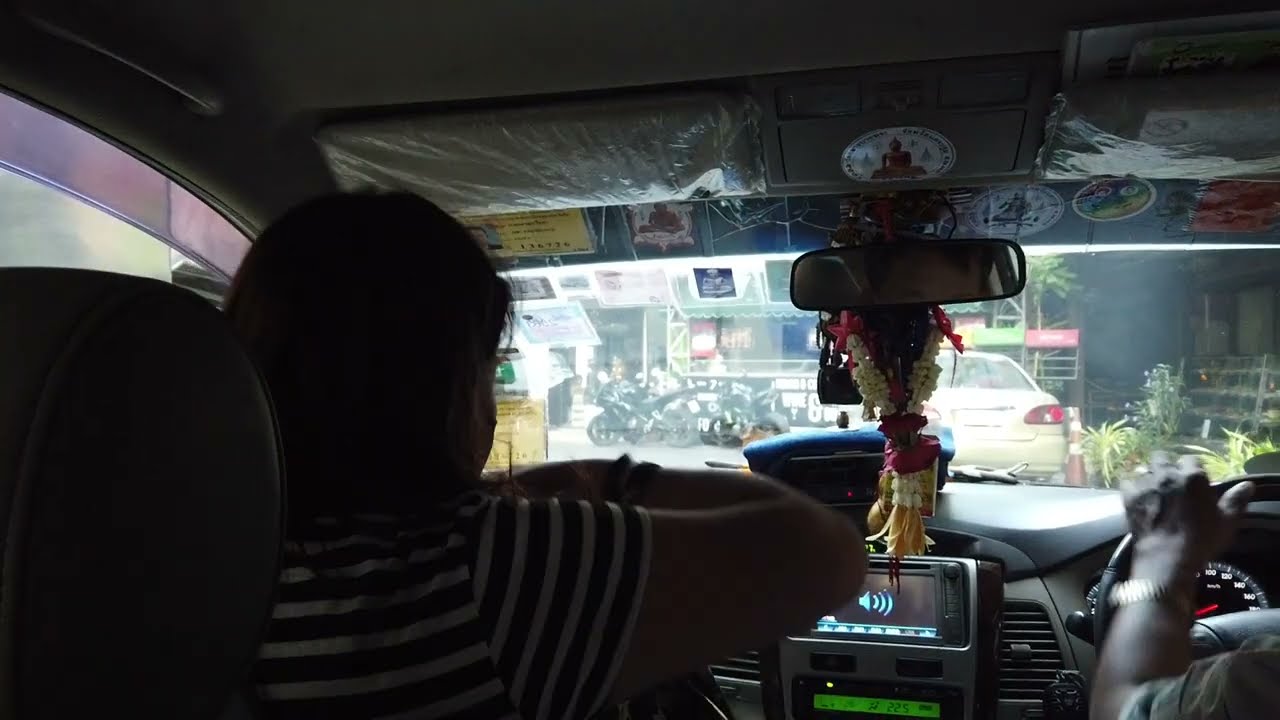In this daytime photo taken inside a car from the back seat, we see two individuals in what appears to be an Asian country. The car has a gray interior with an LED screen displaying an audio icon. The driver, a person with dark skin wearing a watch on their wrist, is on the right side, indicating the car is equipped for left-side driving. Beside the driver sits a female passenger, easily identifiable by her shoulder-length dark hair and black-and-white striped t-shirt.

The image captures a busy street scene through the windshield. Ahead, there's a golden car, and several motorcycles and bicycles are parked in front of stores on a sharp corner. There are trees and weeds visible in the distance, near a wooden hut. The exotic setting is accentuated by cultural elements inside the car—a Buddha sticker on the roof and a rearview mirror adorned with hanging flowers, including lilies and roses. Street signs with Indian writing hint that the location is likely India.